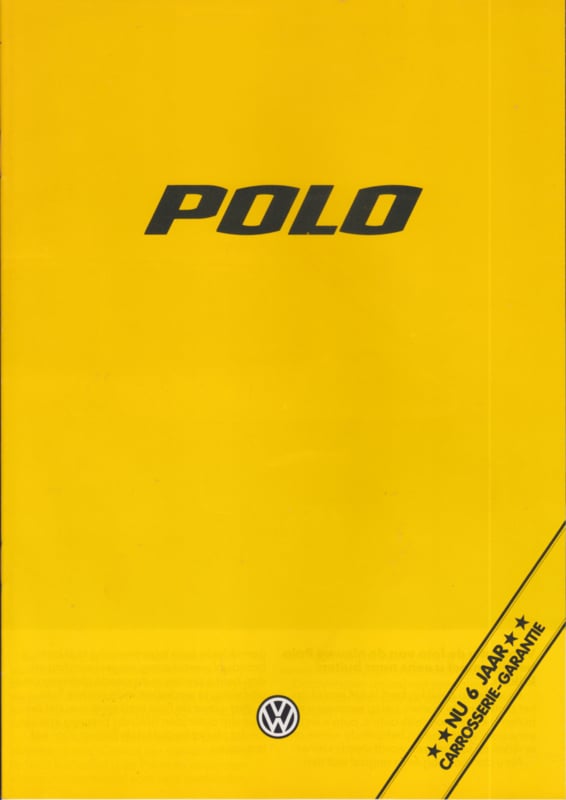The image features a bright yellow background with a gradient that darkens slightly towards an orange hue. Dominating the top center, there is the word "Polo" in large, bold black letters, slightly italicized. Near the center bottom of the image, there's a small Volkswagen logo, comprised of a white "V" above a "W" enclosed in a white circle against a black background. In the lower right corner, a diagonal black banner with stars surrounding the text "NU6JAAR" is present, accompanied by the phrase "Carrosserie Garantie" in black letters. This detailed design suggests it might be the cover of a book or an instruction manual, likely related to a Volkswagen Polo vehicle, possibly indicating a curiosity guarantee or some event associated with the brand.